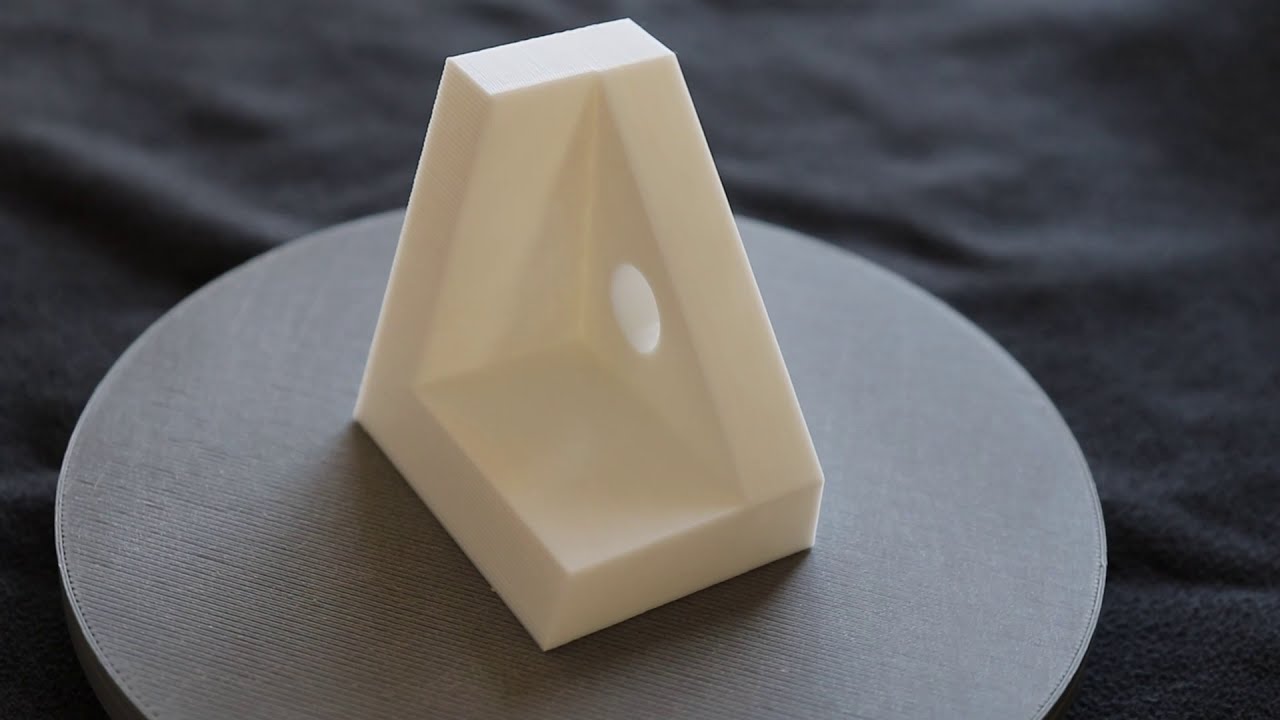The image features a detailed, close-up photograph of an abstract, white 3D-printed sculpture. The sculpture, smooth and synthetic in appearance, resembles the corner of a room; it has one side forming a right triangle with a central circular cutout, while the other two sides are rectangular. The sculpture sits on a dark gray, circular disc surface, which is likely a 3D-printed pad with noticeable horizontal lines and some textural grain. Surrounding this disc is a slightly out-of-focus navy blue or black fabric, possibly a fleece blanket, exhibiting a few wrinkles and stitch patterns. The intricate details of the sculpture, along with the contrast between the white object, the gray disc, and the dark fabric, create a visually compelling and textured composition.